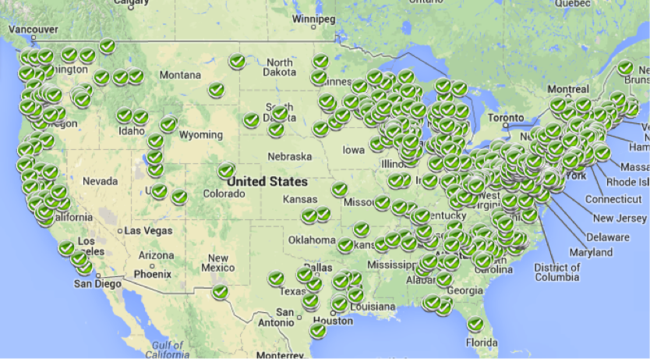This graphic is a detailed map of the contiguous United States, showcasing all the states clearly labeled. The landmass is depicted in a light green hue, while the surrounding oceans are a delicate light blue. Over the map, numerous small green circles adorned with white check marks are scattered, heavily clustered along the East Coast and extending westward to Illinois. The states are labeled in black font at their centers, with additional lines extending out into the Atlantic Ocean to label the smaller eastern states that lack space within their borders. At the top of the map, portions of Canada are visible and labeled, while portions of Mexico are also somewhat labeled. The map includes the prominent title "United States" and provides a comprehensive view of the country's geographical layout.